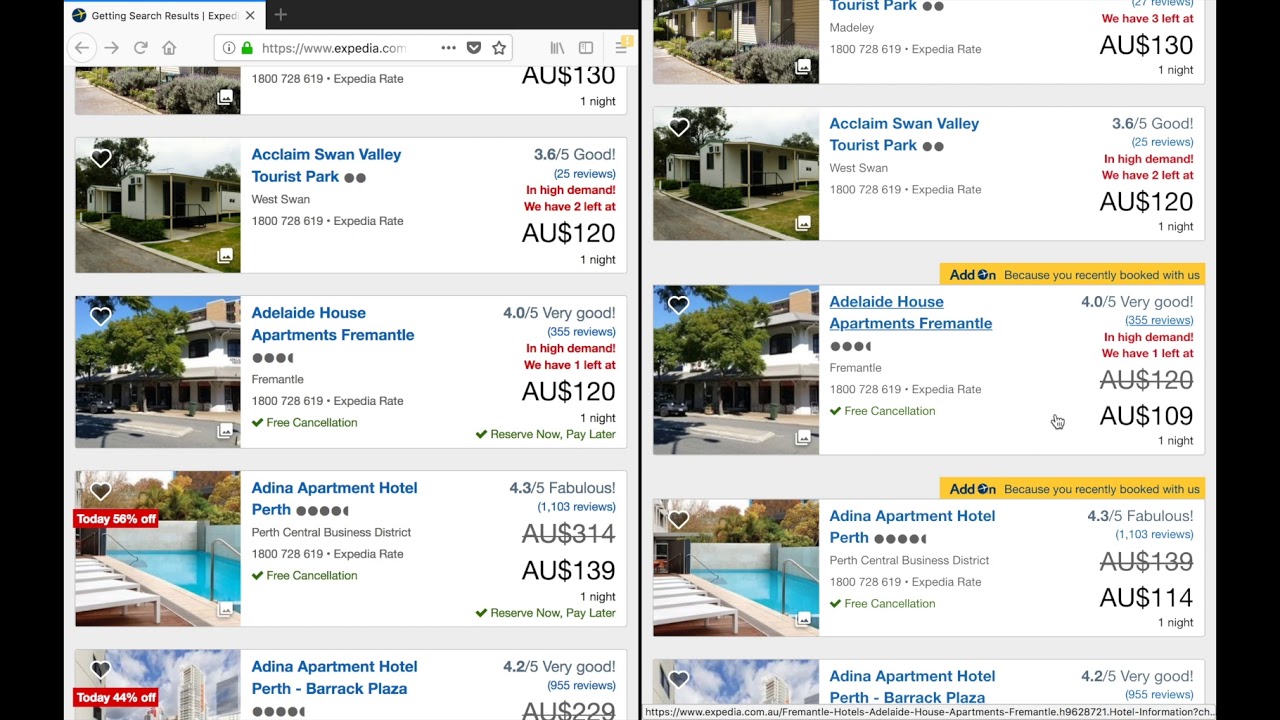**Websites - Search Results for Rentals**

The image under the "Websites" heading displays search results for accommodations available on Expedia, featuring various rental options that seem to emphasize vacation stays, including home purchases and apartments.

1. **Acclaim Swan Valley Tourist Park**: This listing, rated at 3.65 out of 5 stars based on 25 reviews, shows mobile homes highly in demand with only two units left.

2. **Adelaide House Apartments in Fremantle**: Rated 4 out of 5 stars, this highly demanded listing priced at $120 suggests a complex of condominiums or apartments offering comfortable living spaces.

3. **Adina Apartment Hotel, Perth**: Priced at $139 per night, this listing includes the appealing feature of an outdoor pool with lounge chairs, providing a relaxing amenity for guests.

The image features both the Acclaim Swan Valley Tourist Park and the Adina Apartment Hotel side by side, which might suggest a redundancy in the display, but emphasizes the tourist appeal of these rental properties located in attractive areas.